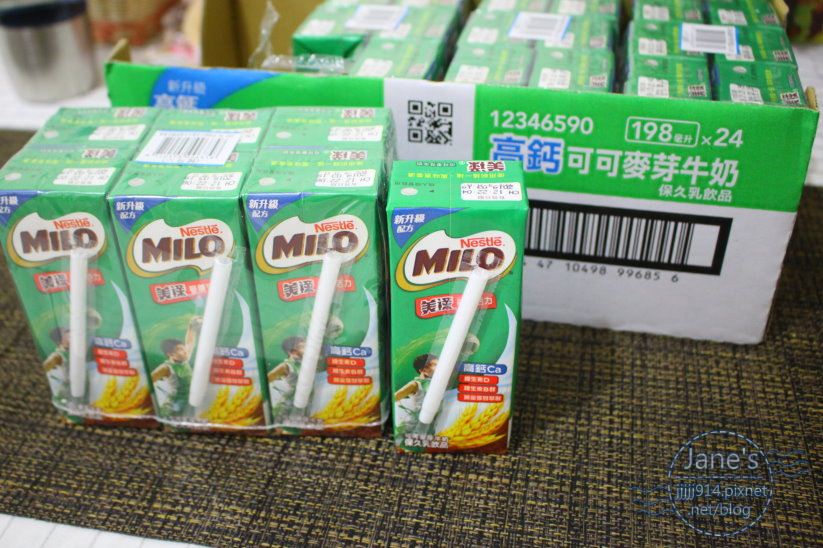The photograph is a detailed, close-up shot of several small cartons of Nestle Milo, a dairy drink primarily marketed towards children. The product is packaged in green cardboard boxes, each equipped with an attached plastic straw. In the foreground, there are seven individual Milo cartons arranged on a burlap mat. Behind them, a larger box containing a 24-count of the same drink is visible, along with several other Milo cartons. The packaging features Asian characters, possibly Japanese or Chinese. The setting appears to be atop a table with a tablecloth, with a trash can and tiled flooring visible in the background. In the bottom right corner of the image, there is a circular watermark reading "Jane's," followed by the URL jjjjj914.pixnet.net/blog.